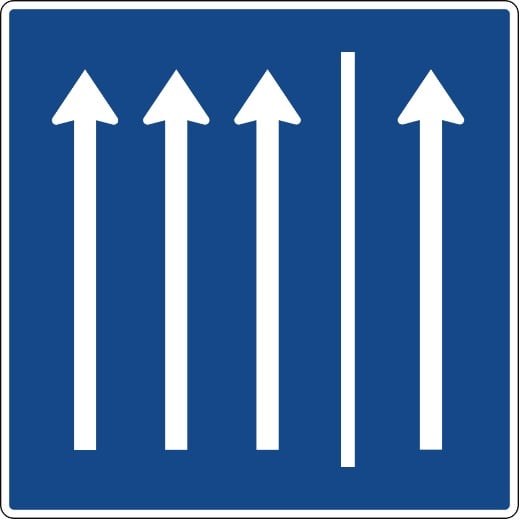The image depicts a traffic sign with a distinctive design. The sign features a black outer border with a white inner border, enclosing a blue square with rounded corners. Inside the blue square, there are four white upward-pointing arrows and a vertical white line. Starting from the left, there are three tall, vertical arrows, each extending from the bottom to the top of the square. Following these arrows, there is a slightly longer, straight vertical white line. To the right of this line, there is another upward-pointing arrow identical to the previous ones. The borders and symbols create a clear and organized layout, potentially indicating different lanes of traffic.